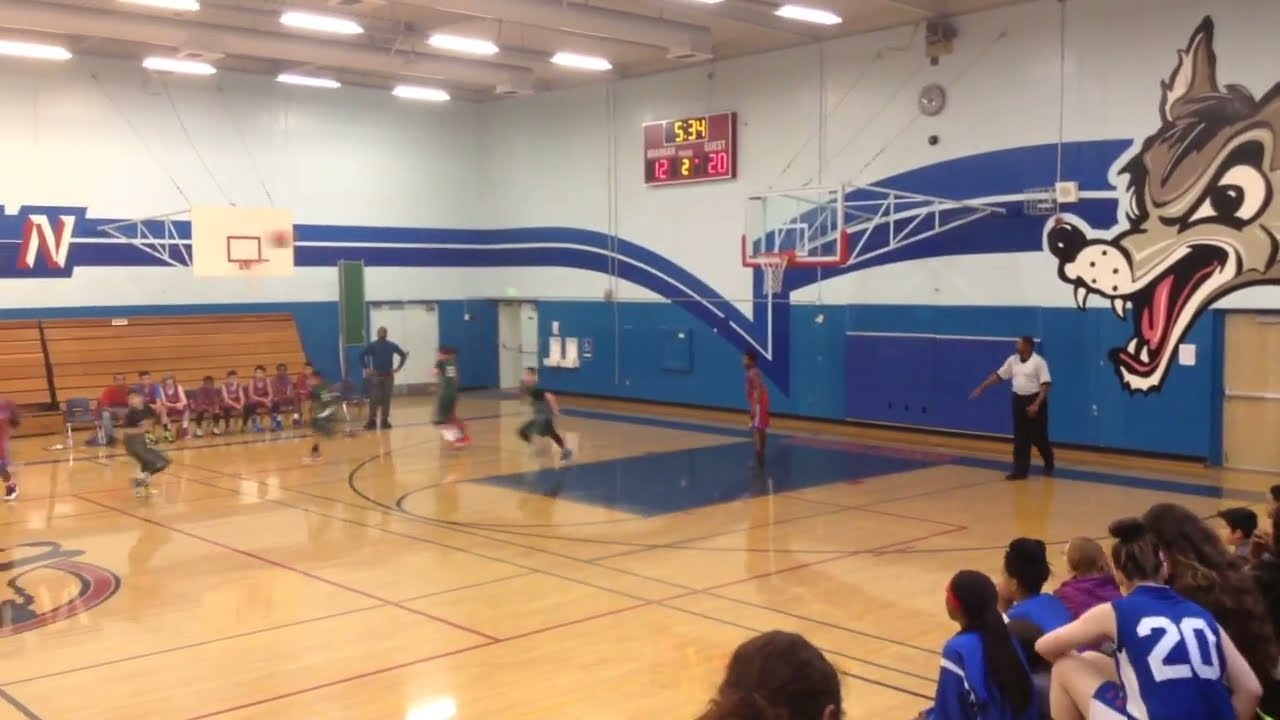The image captures an intense basketball game in a bustling auditorium. Dominating the scene is the wooden basketball court, at the center of which is a striking wolf logo, encircled by red and dark blue colors. Players from two opposing teams, one in dark green and the other in red, are in the midst of heated action. A player from the red team controls the ball at midcourt as teammates and opponents rush towards either side of the play.

In the background, mounted on the wall, is a prominent school logo in blue, red, and white that reads "Sam Brannan," flanked by two suspended basketball backboards and nets on either side. Underneath the logo, wooden bleachers are folded up, emphasizing the space behind the players. On either side of the court, players sit on benches alongside their coaches, near a scorers' table adorned with a red drape, where two officials are seated. The foreground shows the heads of engaged spectators, hinting at the vibrant atmosphere as they eagerly watch the game unfold. The overall scene is rich in detail, showcasing a well-fought match surrounded by the institutional pride of Sam Brannan and the community's support.